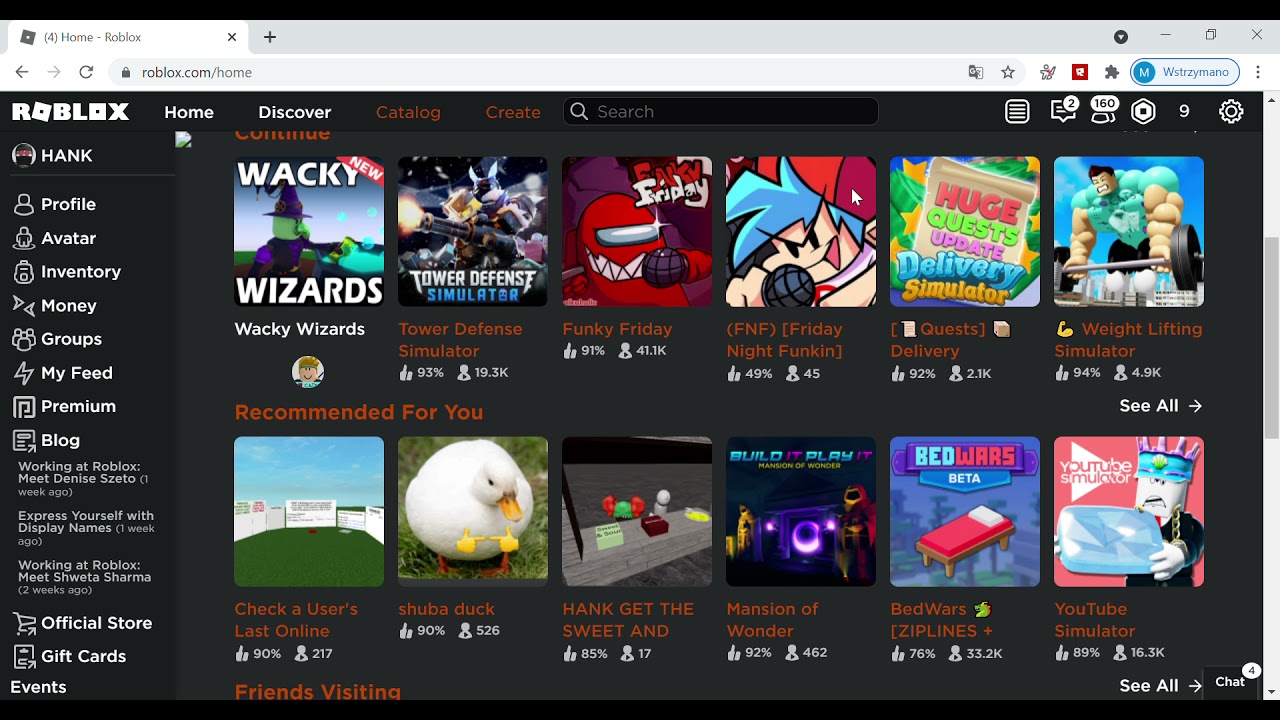The screenshot features the Roblox website's user interface, displayed in dark mode with a black background and white text. At the top of the page, several sections are visible, including 'Home,' 'Discover,' 'Catalog,' and 'Create.' There is also a search bar, icons for unread messages and conversations, and a gear icon for settings.

On the left side of the interface, the user, signed in as 'Hank,' is represented by an avatar resembling a game character. Below the avatar, menu options such as 'Profile,' 'Avatar,' 'Inventory,' 'Money,' 'Groups,' 'My Feed,' and 'Premium Blog' are listed.

The main section of the page showcases various user-created or developer-created games and experiences. These include titles like 'Wacky Wizards,' 'Tower Defense Simulator,' 'Funky Friday,' 'Shoe Bud Duck,' 'Bed Wars,' and 'YouTube Simulator.' The games have a cartoonish and whimsical appearance, indicative of the creative and playful nature of the Roblox platform.